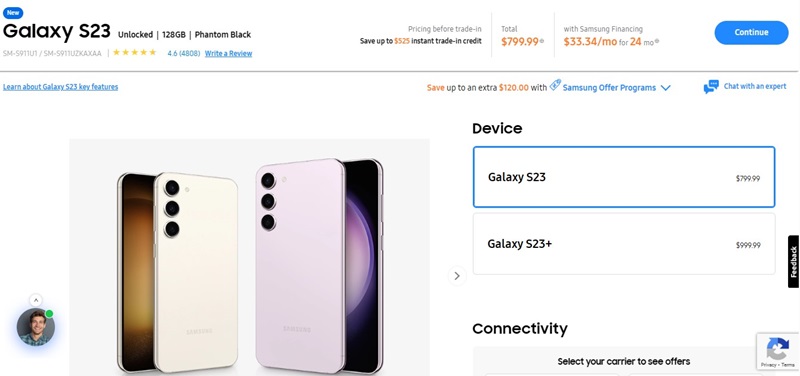This image displays a product page for the Samsung Galaxy S23 smartphone. In the upper left corner, a prominent blue box labeled "New" catches the eye. Directly adjacent, in the upper right section, the text "Galaxy S23" appears just below another blue bubble, indicating various model details: "Unlocked, 128GB, Phantom Black." Below this, a row of five gold stars signifies a user rating of 4.6 based on 4,808 reviews.

The pricing information is detailed beneath the stars, stating that the phone is available for $799.99 prior to any trade-in offers. A note mentions that customers can save up to $525 with an instant trade-in credit. For those opting for financing, payments are broken down to $33.34 per month over 24 months through Samsung financing. A prominent blue "Continue" button is also visible for user interaction.

The middle of the screen showcases different color options for the Galaxy S23, specifically highlighting a white version and a pink version of the phone. Text alongside these images indicates the different models available: the "Galaxy S23" and an option for the "Galaxy S23 Plus."